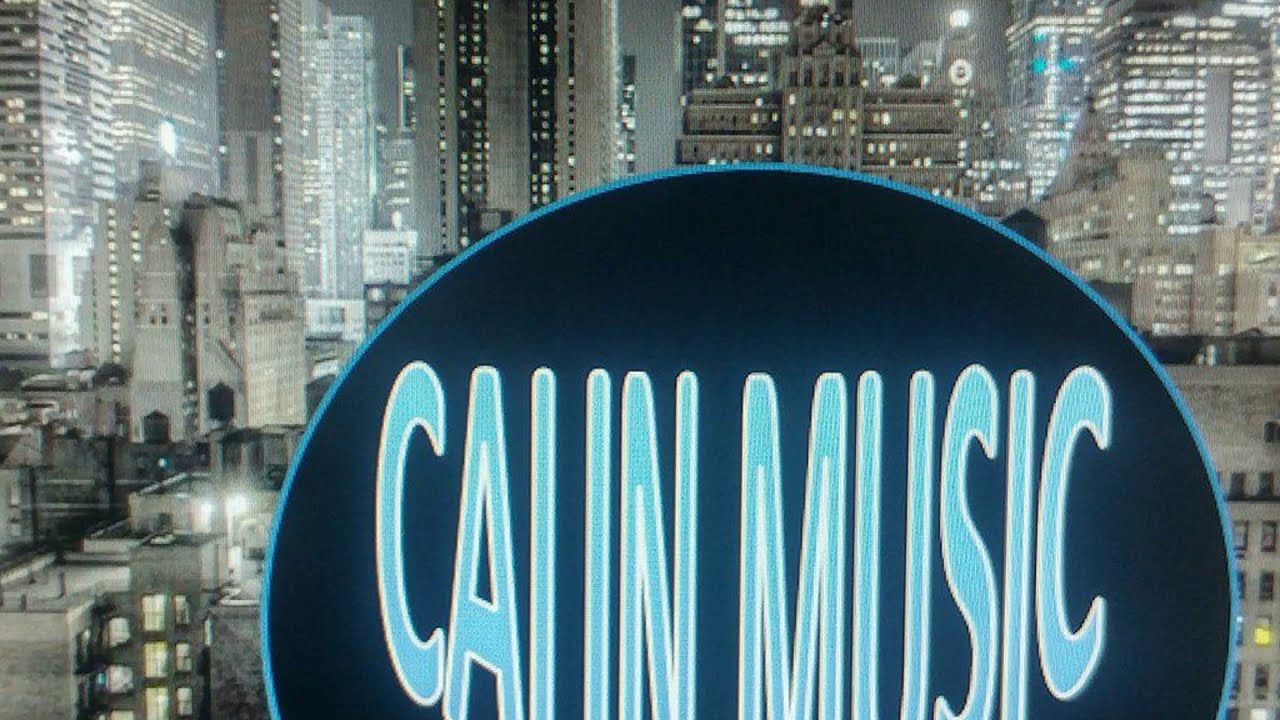The image captures a nighttime cityscape in grayscale with blue highlights, featuring numerous illuminated skyscrapers in the background. In the foreground, there is a large, partially visible circular sign, appearing to be attached to a window. The visible text on the sign reads "CAHN MUSIC" in all capital letters. The outer circle of the sign has a light blue color, while the inner fill is a darker blue. The text "CAHN MUSIC" is outlined in a lighter blue with hints of cream. This juxtaposition of the vibrant blue logo against the grayscale city skyline creates a striking visual contrast, reminiscent of major urban environments like New York City or Tokyo.